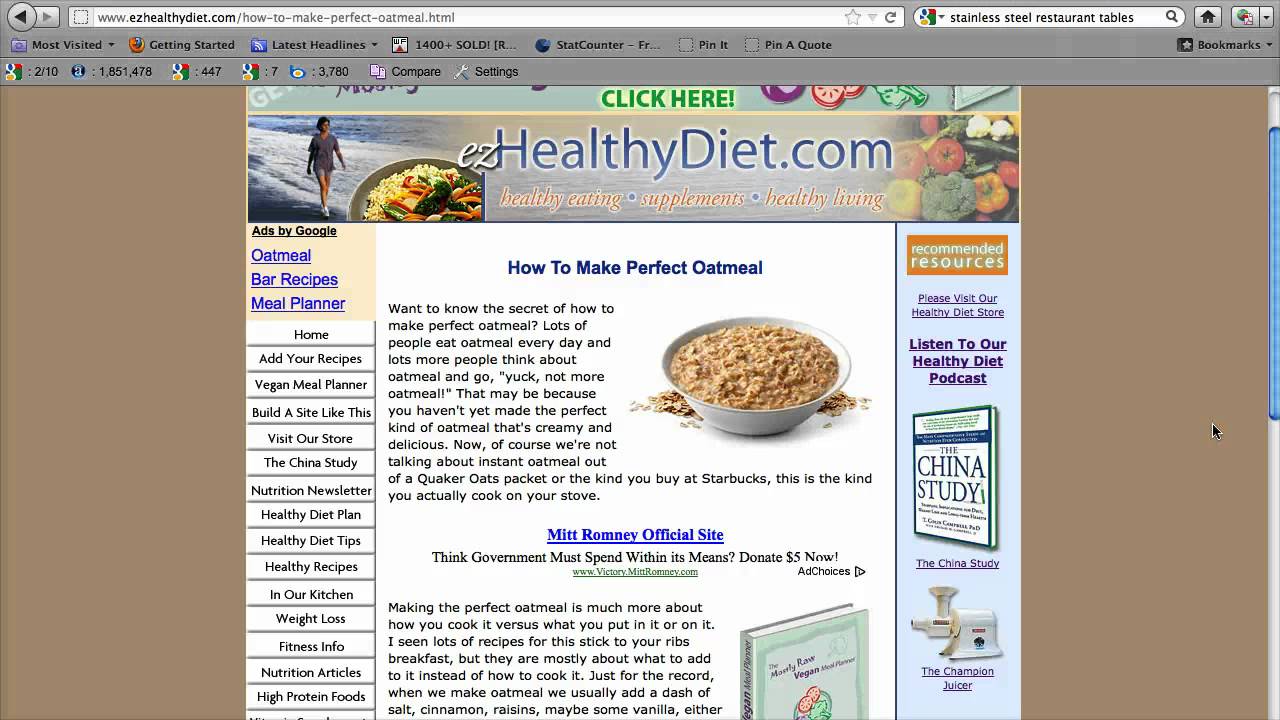This screenshot showcases an outdated browser, possibly from 15 years ago, displaying a similarly aged website, EasyHealthStyles.com, specifically the page "How to Make Perfect Oatmeal". The browser features a gray search bar and bookmark bar at the top. The webpage is distinctly framed by two brown columns on either side, focusing attention on the central content. 

At the very top of the page is the header, prominently displaying "EasyHealthDiet.com". The word "Easy" is in cursive, small, and white, while "HealthDiet.com" is in a larger, blue font. Above this header, a smaller green text prompts visitors to "Click Here." Flanking the header are images: a woman strolling on a beach, a plate of healthy food on the left, and a bowl of assorted vegetables on the right. Beneath the primary header, the description "Healthy eating, supplements, and healthy living" is displayed, separated by blue bullets, in a subtle orange or brown font.

The left column of the site is filled with numerous navigation links, approximately 15, directing visitors to various sections such as "Home", "Add Your Recipes", "Vegan Meal Planner", "Visit Our Store", "HealthyDiet.com", "Healthy Diet Plan", "Healthy Diet Tips", and more. 

The article itself is titled "How to Make Perfect Oatmeal" and opens with an image of a bowl of oatmeal. Alongside the main content, the right column contains advertisements for health-related books and products. Notably, an advertisement for Mitt Romney’s official site is embedded within the article text, standing out amidst the extensive guide on oatmeal preparation.